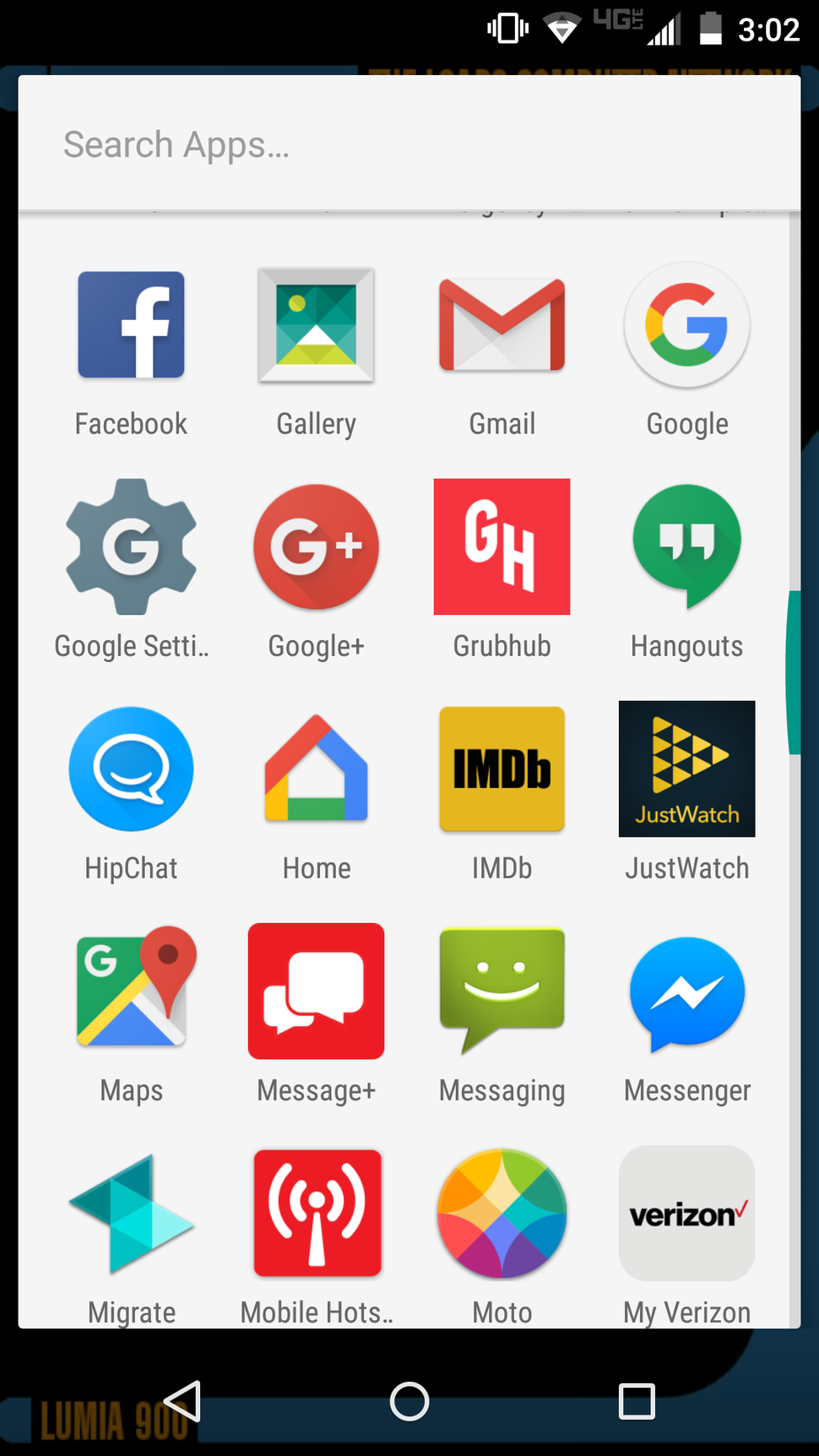The image appears to be a screenshot of an Android phone's home screen. At the very top, various status icons indicate the phone's connectivity and status: a signal strength icon, a 4G LTE symbol, and a low battery warning. The clock in the top-right corner displays "3:02." Below the status bar, there's a search bar labeled "Search apps."

The home screen features a grid of apps arranged in five rows. The visible app icons include Facebook, Gallery, Gmail, Google, Google Settings, Google+, Grubhub, Hangouts, HipChat, Home, IMDB, Just Watch, Maps, Message+, Messaging, Messenger, Migrate, Mobile Hotspot, Moto, and My Verizon.

At the bottom of the screen, the faint label "Lumia 900" suggests the phone's model, though this is likely an error since Lumia 900 is a Windows phone, not an Android. The navigation buttons at the bottom consist of a triangle, circle, and square, typical of Android devices. The background of the app grid is white, contrasting with the black status bar at the top.